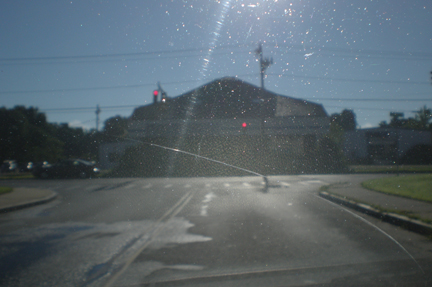The photograph captures a seemingly mundane yet detailed scene taken from inside a car, looking out through the slightly dirty windshield adorned with wiper streaks and nicks. It showcases a bright, cloudless blue sky, abundantly lit from above but without the sun visible, suggesting a sunny day. The two-lane road stretches out ahead with a clear center line, flanked by neatly manicured green lawns and sidewalks on both sides.

The car in view appears to be slowing down or stopped at a red light, emphasizing a sense of motion paused. Directly ahead, a one-story, dark-colored building with a peaked roof stands at the end of the road, creating a T-intersection forcing traffic to turn left or right. The structure is nondescript but has a storefront appearance, with red traffic lights hanging above it. Behind the building, electrical wires stretch across the scene, and to its left is a small parking lot with a few parked cars and some surrounding trees.

The road surface is wet, hinting that it might have just rained, adding reflections and glare that obscure some details. Overall, the image captures an ordinary moment made intriguing by the interplay of light, shadow, and reflections.